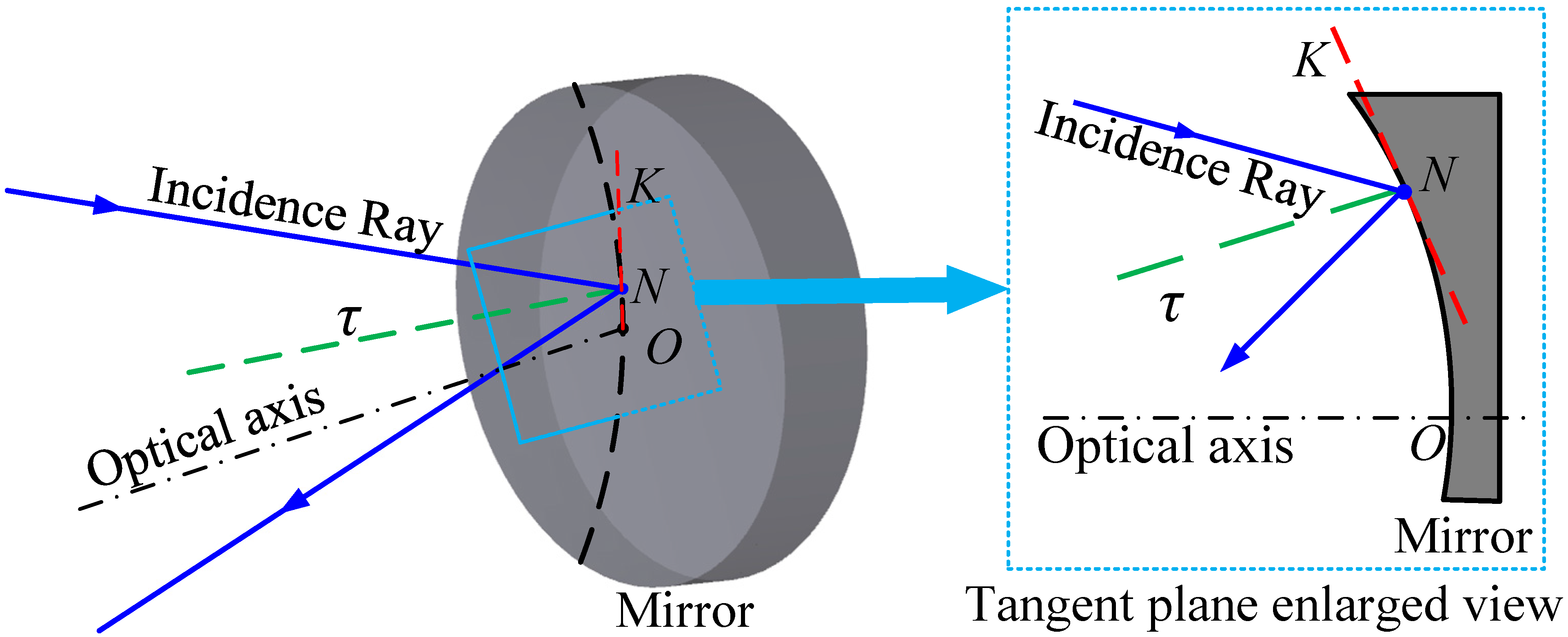The detailed technical illustration showcases an optical axis and the incidence ray interacting with a concave mirror. The main diagram situates the concave side of the mirror on the left, detailing the angles of the incidence ray as it intersects with the optical axis at the center of the concave surface. Key points such as K, N, O, and π are labeled clearly. 

To the right, a magnified section of the mirror, highlighted in blue and boxed in, provides a closer view of the interactions at points K, N, and O. The optical axis and incidence ray are depicted with blue arrows, illustrating their precise trajectory and how they reflect off the mirror.

Additionally, a secondary diagram offers a colored, side-view perspective of the mirror, emphasizing the tangent plane where the incident ray and optical axis are also represented. In this view, the K, N, and O points are marked on a curved line with red dashes, while the optical axis and incident rays are consistently shown through blue arrows, further clarifying the light's path and angles of incidence. The diagram is comprehensively labeled to enhance understanding of the optical interactions at play.